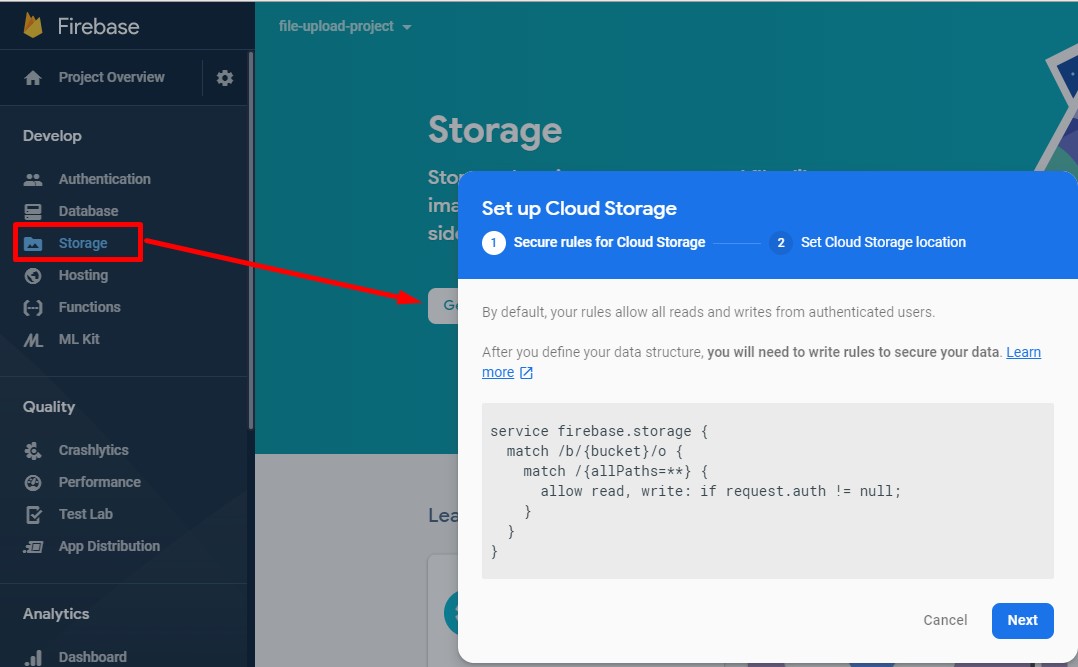The image displays a web page from Firebase, characterized by a navy blue vertical ribbon on the left side of the screen. At the top of this ribbon, the word "Firebase" is displayed alongside a fire icon. Below this, the ribbon features "Project Overview" in white text, flanked by a home icon to its left and a settings gear icon to its right.

Further down the ribbon, there is a vertical list of categories starting with "Develop," under which are listed: Authentication, Database, Storage, Hosting, Functions, and ML Kit. Notably, "Storage" is highlighted with a red box and an accompanying red arrow pointing towards the main section of the page.

In the primary display area of the screen, there is a white box containing green text; however, this box is partially obscured by a pop-up overlay. This overlay, which has appeared on top of the main content, is intended for configuring cloud storage settings and contains a substantial amount of data and information.

Additionally, beneath the Develop categories on the ribbon are Quality categories: Crashlytics, Performance, Test Lab, and App Distribution, followed by Analytics. Despite the overlay, the word "Storage" is visible in white text on a green background in the main screen area, though further content is hidden beneath the pop-up setup box.